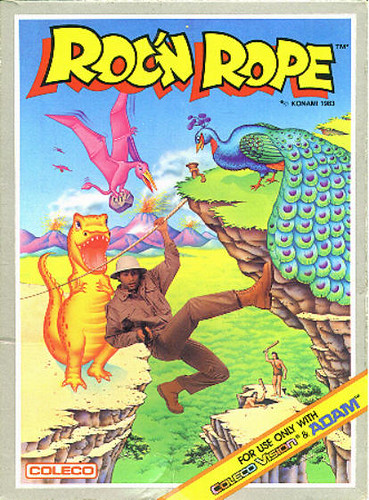This image features the front cover of the game box for "Rock 'n Rope," a title designed for use with ColecoVision and the Atom. Prominently displayed at the bottom left is the Coleco brand logo. The main visual depicts an adventurous man in a safari hat, dressed in a tan shirt, pants, and boots, swinging from a rope in a bold and dynamic pose. Behind him, a bright yellow dinosaur perches menacingly on a cliff. Above, a pink pterodactyl soars through the sky with a rock marked by the number 5 clutched in its talons. Below, on a separate cliff, a caveman figure wielding a stick appears poised to strike another caveman who is struggling to ascend. Adding to the vibrant chaos, a peacock is visible in the top right corner of the scene.